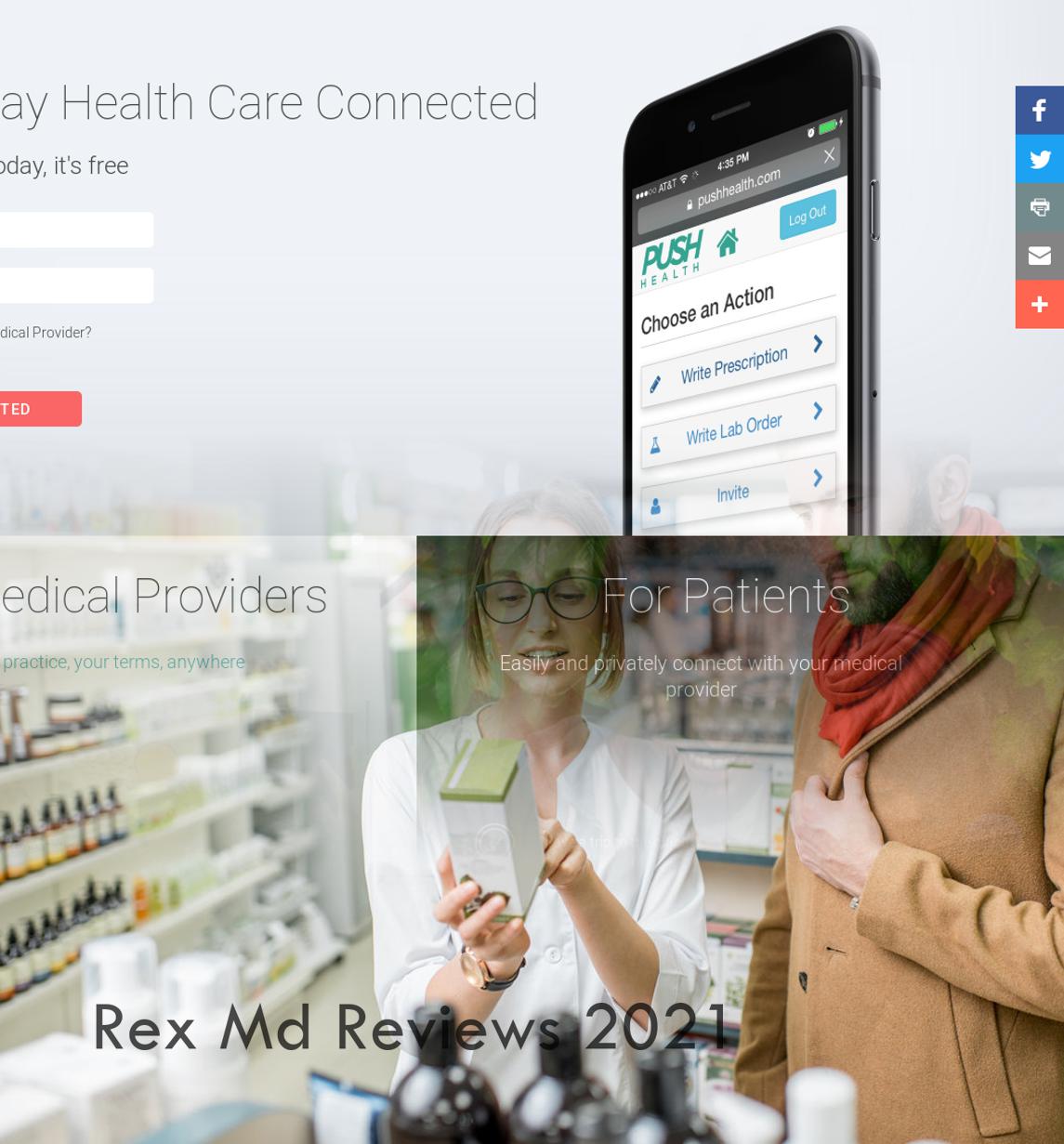In this image, we see a composite layout set against a light gray background. At the top, there is a color photo of a black cell phone facing slightly to the west. The screen of the cell phone is on and displays the Push Health application interface, presenting options such as "Choose an Action," "Write Prescription," "Write Lab Order," and "Invite." At the upper left corner of the phone screen, there are the words "Health Care Connected" accompanied by two white form boxes.

Below this, there is another photograph depicting a woman and a man standing in what appears to be a pharmacy environment. The woman, who has short blonde hair, is wearing a white shirt and is holding a box that both individuals are examining. The man, who is turned sideways, is dressed in a camel-colored jacket and an orange scarf. Both appear focused on the contents of the box. Beneath this photo, in gray block text, the words "RexMD Reviews 2021" are prominently displayed.